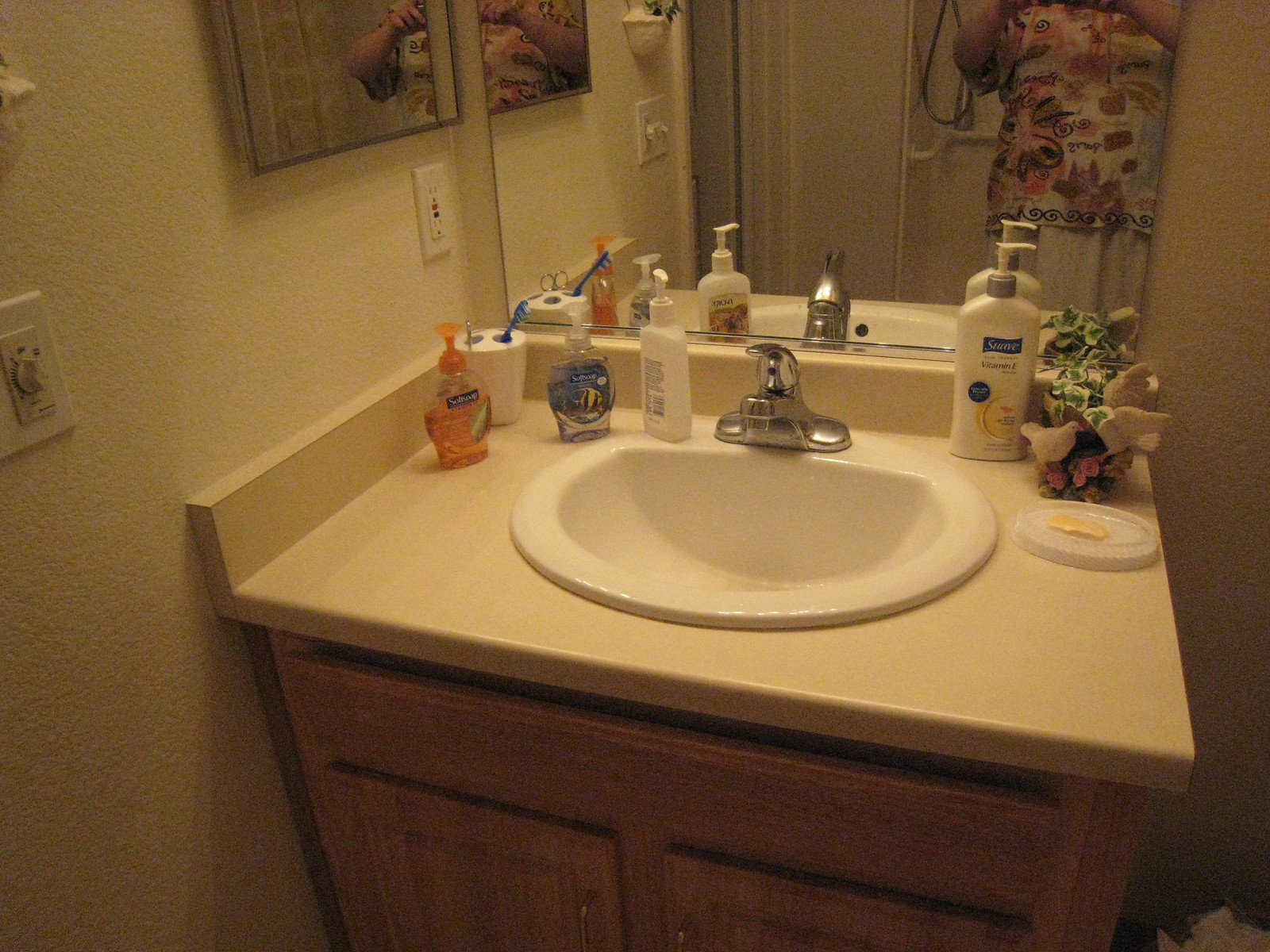In the image, we see a well-organized bathroom sink area featuring a simple white ceramic sink paired with a sleek silver faucet. Mounted just behind the sink is a plain mirror reflecting the scene and part of the photographer. The countertop displays a white container designed to hold toothbrushes, with a blue toothbrush placed in one of the two openings.

Adjacent to the toothbrush holder are two containers of hand soap—one orange and the other a translucent blue. There are also two lotion containers; one is from the brand Equate, and the other from Suave. 

To the right of the sink sits a white soap dish holding a well-used bar of yellow soap. Above this, a small decoration of green leaves adds a touch of nature to the setting.

Visible in the mirror is a person wearing a floral shirt whose arms are partially in the frame, holding the camera to capture this meticulously arranged bathroom sink.